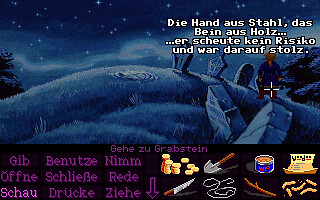The image is a horizontal screen capture from an old point-and-click adventure game, written in what appears to be German. The main scene shows a nighttime setting with a dark blue sky sprinkled with white stars and some horizon clouds, depicting a hill with pentagonal-shaped tombstones or graves. Towards the right-hand side of the hill, there's a squatting or sitting figure with white text in German floating above him that reads, “Die Hand aus Stahl, das Bein aus Holz, er schultet kein Recycle und war dorant Stahls.” The overall scene has a solemn, eerie atmosphere. The bottom portion of the screen is black with three rows of purple German text on the left and a 2x4 grid of inventory items on the right. The inventory items include a pile of gold coins, a shovel, a jar of food, a decree or deed, a steak knife, a wire, a twig, and worms. The entire setup strongly evokes the feel of vintage adventure games, with detailed visual and textual elements enhancing the immersive experience.